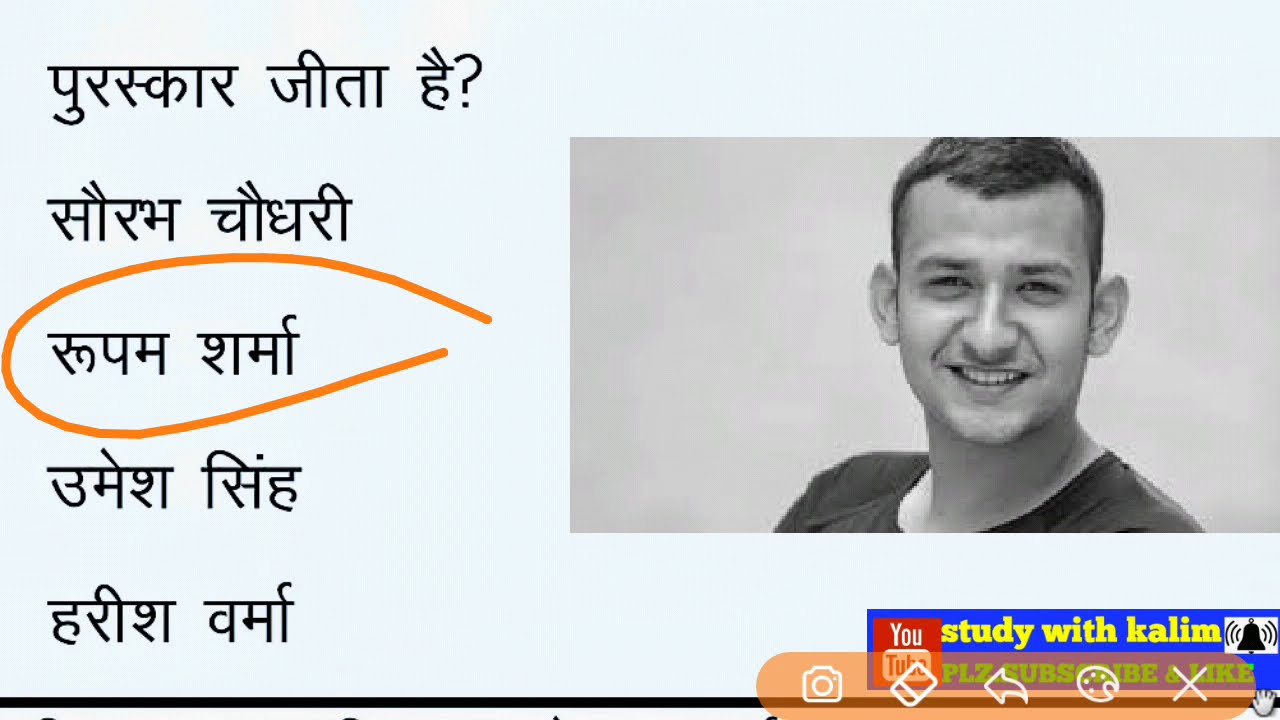The image appears to be a graphic designed for YouTube or an online advertisement, featuring a light blue background. On the right side, there is a rectangular cutout portraying a smiling young gentleman with neatly cropped short dark hair and prominent ears wearing a scoop neck t-shirt. He is looking directly at the viewer, and there’s a visible upbeat expression showing the top row of his teeth.

Positioned below his photo, there is a blue banner that reads "YouTube" in larger text, followed by "Study with Kaleem," with "Study with Kaleem" highlighted in yellow. Underneath, in green text, it says "Please subscribe and like," potentially urging viewers to engage with the content. Overlaying this blue rectangle is a semi-transparent orange oval containing various icons such as a camera, eraser, reset arrow, artist palette, and an X symbol.

On the left side of the image, there are five rows of text written in a foreign language, possibly Arabic or Hindi. The third line of this text is circled in orange, emphasizing that particular section. Overall, the graphic utilizes a mixture of visual and textual elements to convey its message effectively.